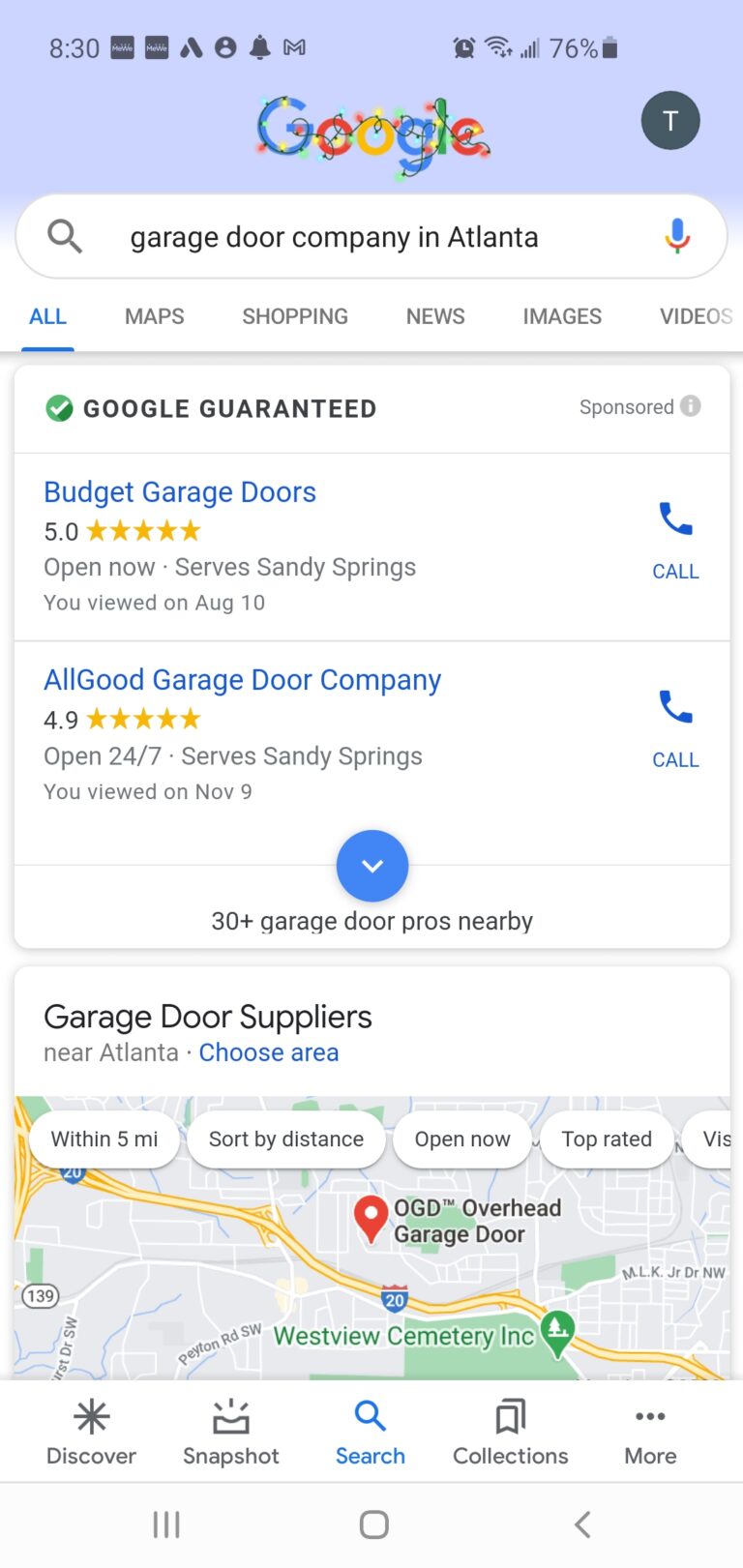The image displays a screenshot from a smartphone. The phone has a tall, rectangular shape, indicative of a typical mobile device. The background color is a very light blue. At the top left corner of the screen, the time is shown as 8:30. Moving across the top, various icons are visible, including a 76% battery life indicator, approximately three bars of Wi-Fi signal strength, and a notification that the volume is turned up.

On the webpage, the user is on the Google search engine home page. The search query at the top reads, "Garage Door Company in Atlanta." Directly below, the screen shows that Google has provided two sponsored results under the "Google Guaranteed" label: "Budget Garage Doors" and "Alley Good Garage Door Company."

Further down, the screen displays a section titled "Garage Door Suppliers," accompanied by a map pinpointing the location of "OGD Overhead Garage Door."

Overall, the detailed view presents an organized search result with specific companies listed as reliable options, alongside a helpful regional map for additional context.